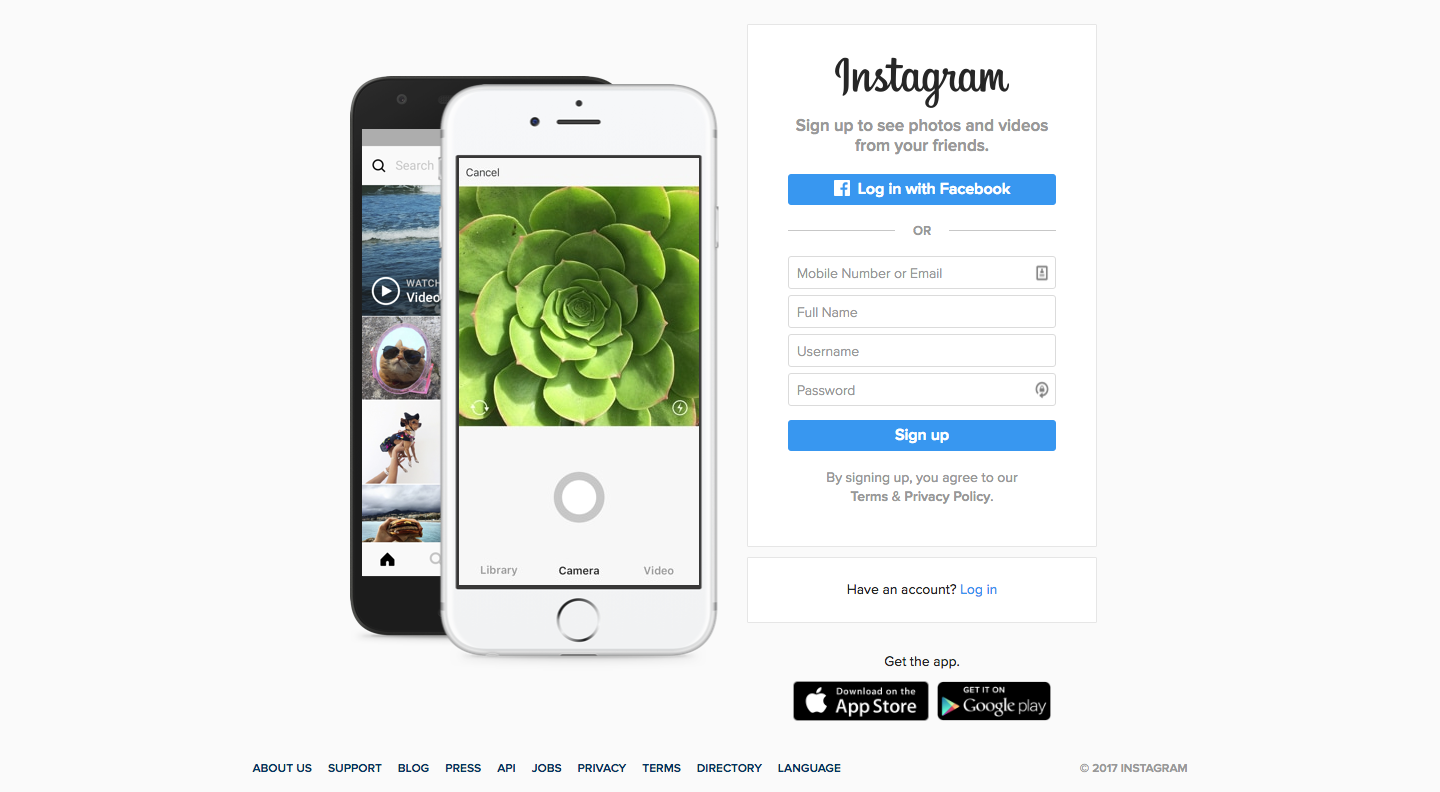This is a cropped screenshot of the Instagram app signup page. On the left side of the image, there are two smartphones displayed. One phone is black, and the other is white, with the white phone angled slightly towards the front right of the black phone. On the right side of the image, there is a large white box with "Instagram" written at the top in bold, black cursive letters. Below the Instagram logo, in small black text, it reads: "Sign up to see photos and videos from your friends." Underneath this prompt, there's a prominent blue button labeled "Log in with Facebook." Below the Facebook login option, in small grey letters, it says "or," followed by fields for entering a mobile phone number or email, full name, username, and password. At the bottom of these input fields, there is a large blue button marked "Sign up." The very bottom right corner of the screen features the App Store and Google Play logos, indicating where the app can be downloaded.